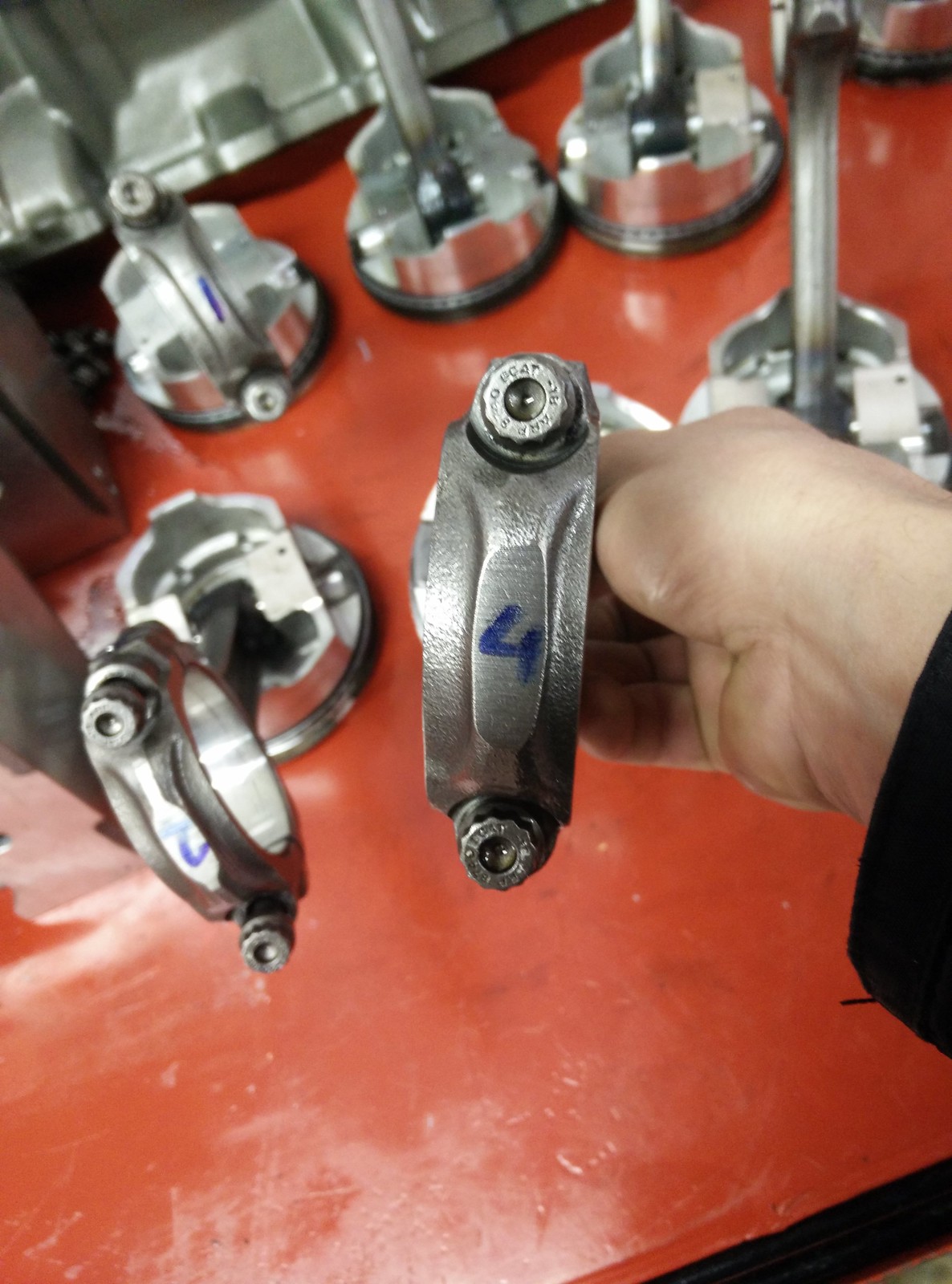The photograph captures six identical metallic tools or instruments, each featuring a silver hue with a base possibly made of darker rubber. These tools are lined up in two rows of three on a bright red, flat work surface. Each tool has a cylindrical component, and the one in the middle of the front row is being held by a person's right hand. This hand, emerging from the right side of the image, has a black sleeve extending to the wrist and belongs to a white individual. The tool being held has two screws—one on the top and one on the bottom—and bears the number four written in blue marker. Occasionally, other tools also display numbers written in blue, such as a one and a possibly five.